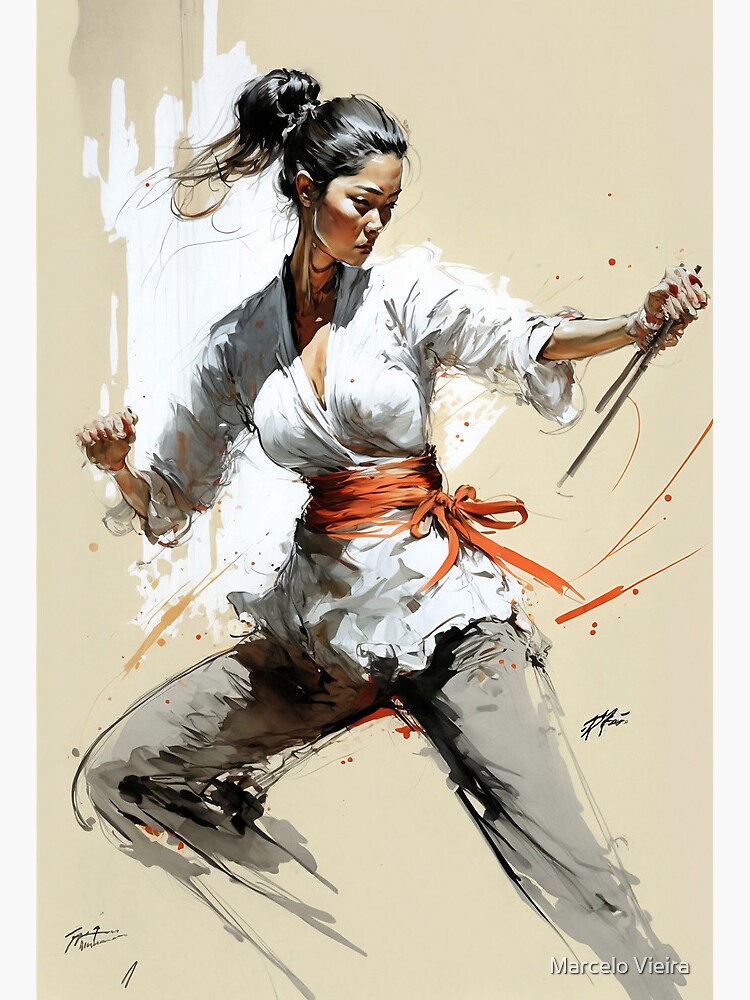This digital illustration, blending sketching and painting techniques, depicts an Asian female martial artist poised in an action stance against a pink-toned background. The subject, with long black hair pulled back into a ponytail, exudes intensity and determination. She is adorned in traditional martial arts attire, featuring gray pants and a white karate gi, secured with a distinct sash that varies in color as described—from orange to red and green. In her hand, she holds an indistinguishable martial arts tool. The image is framed vertically and features the artist's signature "Marcelo Vieira" at the bottom.